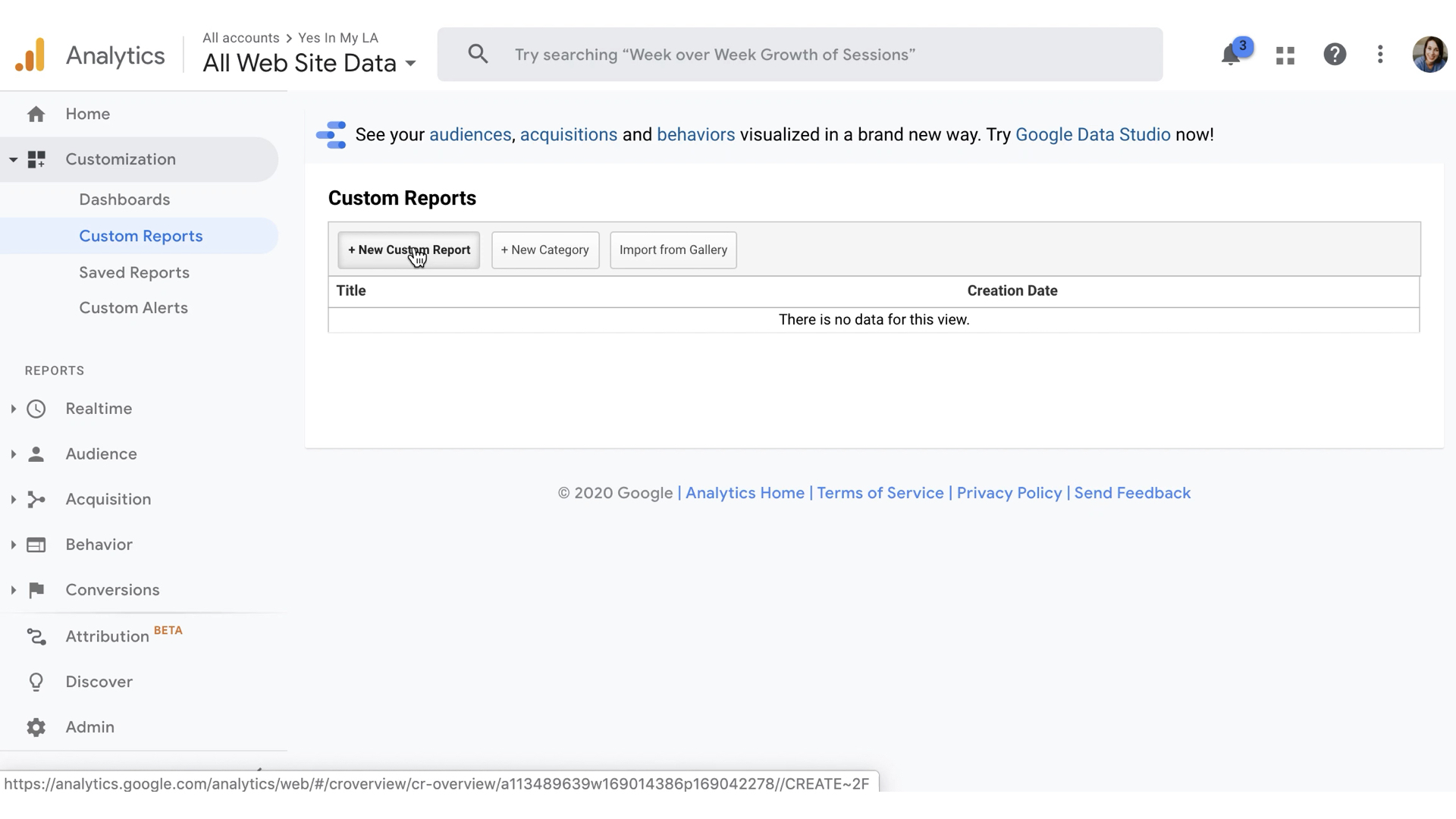The image depicts a comprehensive view of a Google Analytics web page. At the top, there is a header that prominently displays the word "Analytics" accompanied by a sequence of colored indicators – a yellow dot, an orange dot, an orange-yellow line, and a white-orange-yellow line. Next to this, "Analytics" is written again with a capital "A," followed by a small vertical line and the phrase "All Accounts" with an arrow pointing to the right. To the right, the text "Yes in my LA" is visible.

Beneath this header, in bold black print, the page lists "All Website Data" accompanied by a downward-facing arrow. Below this is a gray band containing a search bar featuring a gray magnifying glass icon and the placeholder text "Try searching 'week-over-week growth of sessions'."

To the right of the search bar, several icons are displayed:
- A bell with a blue circle showing the number three inside it.
- A grid of four squares with a plus sign in the center.
- A gray circle with a white question mark.
- A vertical ellipsis (three dots arranged vertically).
- A circular user avatar.

Towards the left side of the page, a sidebar menu lists several items:
- Home
- Customization
- Dashboards
- Custom Reports
- Saved Reports
- Real-time Alerts
- Reports
  - Real-time
  - Audience
  - Acquisition
  - Behavior
  - Conversions
  - Attributions (with "beta" in orange)
- Discover
- Admin

In the center of the page is a promotional banner that reads, "See your audiences, acquisitions, and behaviors visualized in a brand new way. Try Google Data Studio now." Below this banner are options for:
- Custom Reports
- New Custom Report
- New Category
- Import from Gallery

Additionally, the page displays headers for "Title" and "Creation Date," followed by a message indicating, "There is no new data for this view."

At the bottom of the web page, the footer includes standard links: "Google Analytics Home," "Terms of Service," "Privacy Policy," and "Feedback," marked for the year 2020.